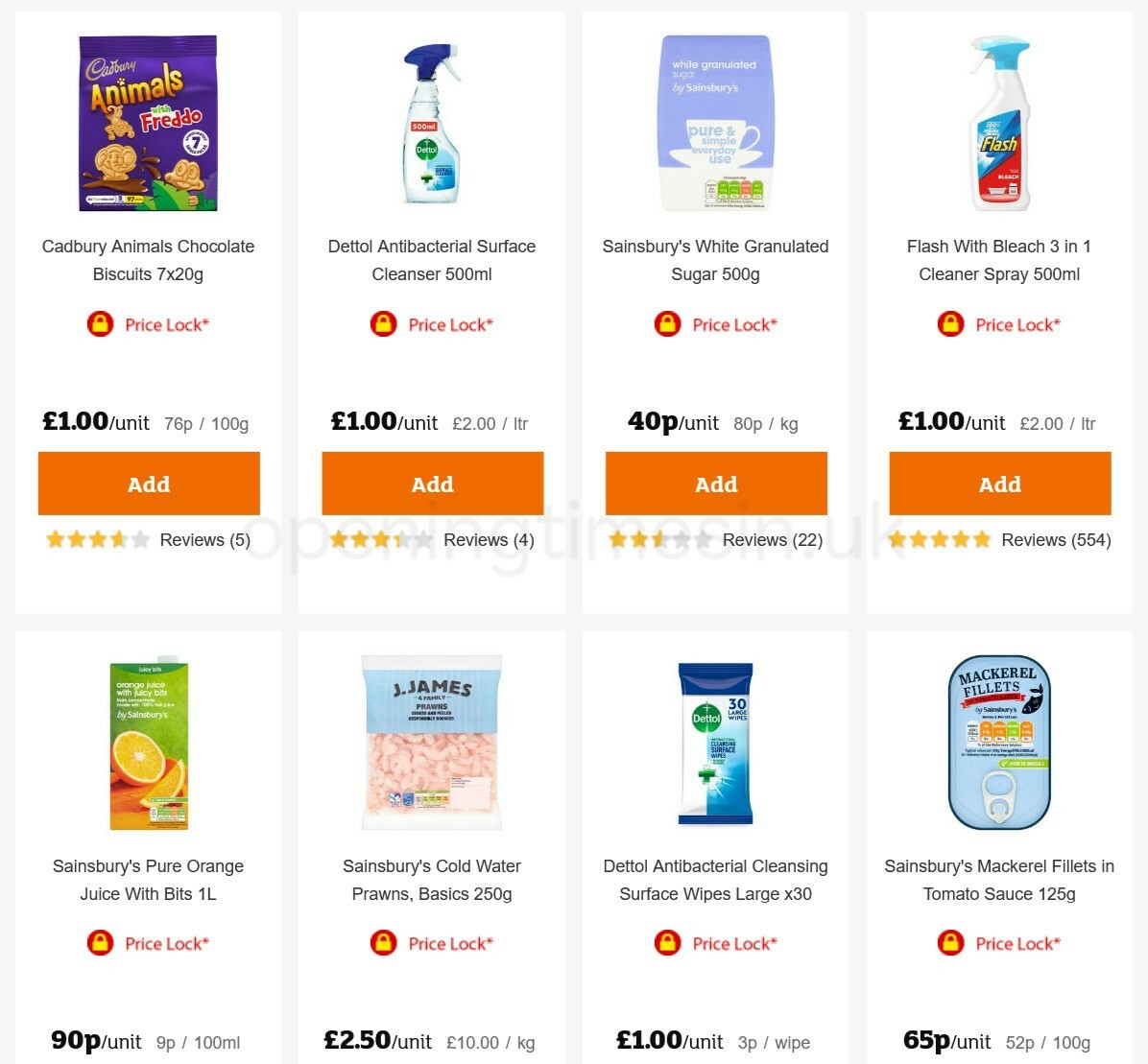Here's a more detailed and cleaned-up caption for the image:

---

The shopping page showcases eight items arranged in two rows, with four items on top and four items below. Each item features an "Add" button for easy addition to the cart, indicated by a prominent orange button with the word "Add" in white.

1. **Cadbury Animal Chocolate Biscuits (7 x 20g)**:
   - Price: £1.00 per unit, £0.76 per 100g
   - Rating: 3.5 stars from 5 reviews
   - Features an "Add" button.

2. **Dettol Antibacterial Surface Cleaner (500ml)**:
   - Price: £1.00 per unit, £2.00 per litre
   - Rating: 3.5 stars from 4 reviews
   - Features an "Add" button.

3. **Sainsbury's White Granulated Sugar (500g)**:
   - Price: £0.40 per unit, £0.80 per kg
   - Rating: 2.5 stars from 22 reviews
   - Features an "Add" button.

4. **Flash with Bleach 3-in-1 Clean Spray (500ml)**:
   - Price: £1.10 per unit, £2.20 per litre
   - Rating: 5 stars from 554 reviews
   - Features an "Add" button.

Each item has a clear rating and price per unit, helping customers make informed decisions based on cost and reviews.